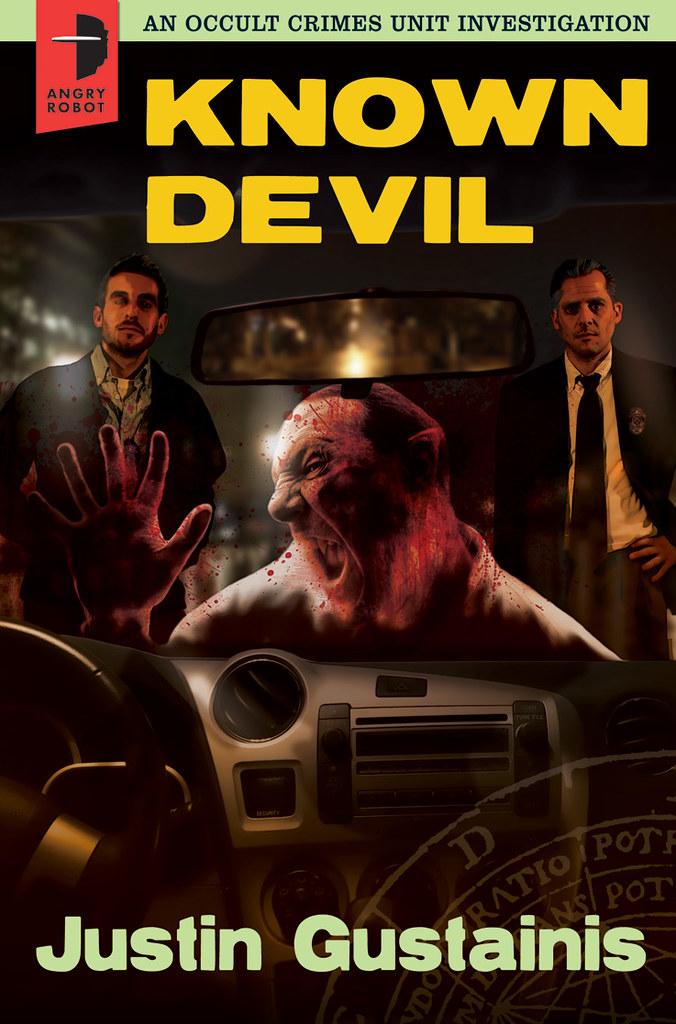This poster, likely a cover for a horror-themed comic book, DVD, or video game, is titled "Known Devil," displayed prominently in big yellow letters. The background features a distressed, possibly demonic, figure pressing his cheek and one bloody hand against the windshield of a car. This creature has pointed ears and a grotesque, distressed expression, suggesting a scene filled with horror and violence. Behind this creature stand two men in suits, who appear to be detectives, remaining strangely calm in the midst of the chaos. At the top of the poster, a light green horizontal strip reads "An Occult Crimes Unit Investigation," and to the top left is the logo for Angry Robot, depicted as a red and black robot face. The author, Justin Gustines, is credited at the bottom of the poster in light green lettering.